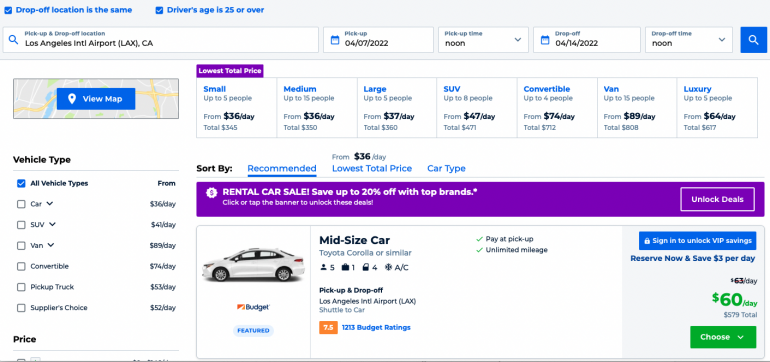Here’s a highly detailed and clean caption for the given image:

---

**Rental Vehicle Details at Los Angeles International Airport (LAX)**

**Pickup and Drop-off Information:**
- **Location:** Los Angeles International Airport (LAX), California
- **Pickup Date:** 04/07/2022 at 12:00 PM
- **Drop-off Date:** 04/14/2022 at 12:00 PM

**Vehicle Types and Prices:**
- **Car:** $360 per day
- **SUV:** $41 per day
- **Van:** $89 per day
- **Convertible:** $74 per day
- **Pickup and Drop-off:** $53 per day (optional)

**Vehicle Size Options:**
- **Small:** Up to 5 people
- **Medium:** Up to 15 people
- **Large:** Up to 5 people
- **Light:** Up to 8 people
- **Luxury:** Up to 5 people

**Sorting Options:**
- **Recommended Age:** Starting from $360 per day
- **Lowest Total Price:** By car type

**Highlighted Properties:**
- **Property 2:** Rental, car sale with savings up to 20%
- **Property 3:** Features for budget, new size cars like Toyota Corolla or similar; seats up to 5 people, accommodates 1 briefcase, 4 doors, available for pay at pickup with unlimited mileage.

**Price Summary:**
- **Rental Rate:** $63 per day, with possibilities to save $3 per day when you sign in to unlock VIP savings

**Call to Action:**
- **Button:** "Choose" in a green rectangle on a white background

---

This caption provides a clear and structured summary, organizing the information into practical categories while maintaining a high level of detail.